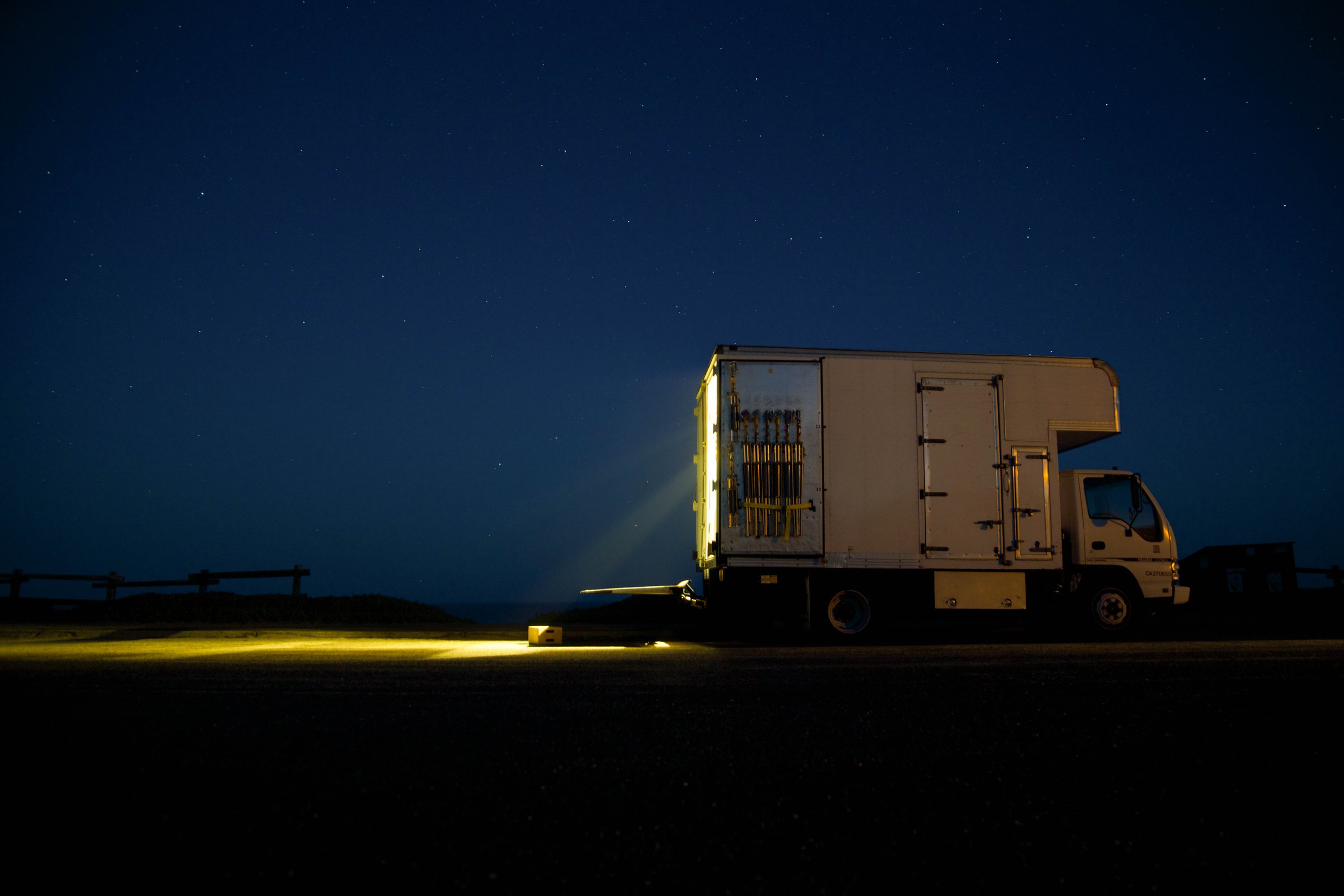This nighttime photograph depicts a white moving truck, reminiscent of a U-Haul, positioned on the right side of the frame. The truck features a cab over the top and a shorter, enclosed trailer-style body, equipped with a hydraulic lift at the back. Dual tires can be seen at the rear, while the front wheels are less visible. The foreground is cloaked in darkness, with the exception of the ground illuminated by a bright light pouring out of the open rear of the truck. This light casts an eerie glow, creating a surreal scene. The sky above is a deep, dark blue, dotted with a few stars, indicating that the sun has set. In the distant background, a vague structure possibly resembling a dock can be discerned, adding a faint contextual layer to the image. No people are present in this photograph, and the overall atmosphere is one of quiet, almost mysterious solitude.